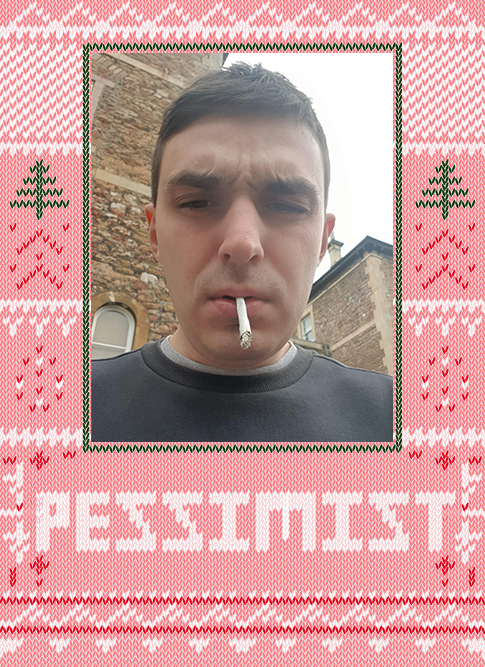The image features a Caucasian man with an angry scowl on his face, smoking a cigarette, and wearing a black shirt. He is positioned in the center, with the backdrop of an old, grey European stone building, under a sky that appears overcast with clouds. The image is framed with a digitally designed pink knitted border that aims to replicate hand-stitched embroidery, giving it a quilt-like appearance. At the bottom of the image, the word "Pessimist" is prominently displayed in white, embroidered-looking text against the pink background. The border also includes Christmas trees along the sides, and the overall color scheme includes pink, white, dark pink, green, red, black, and various shades of brown. This intricate design suggests the piece may be a poster or a greeting card, emphasizing the theme conveyed by the man's expression and the word "Pessimist."